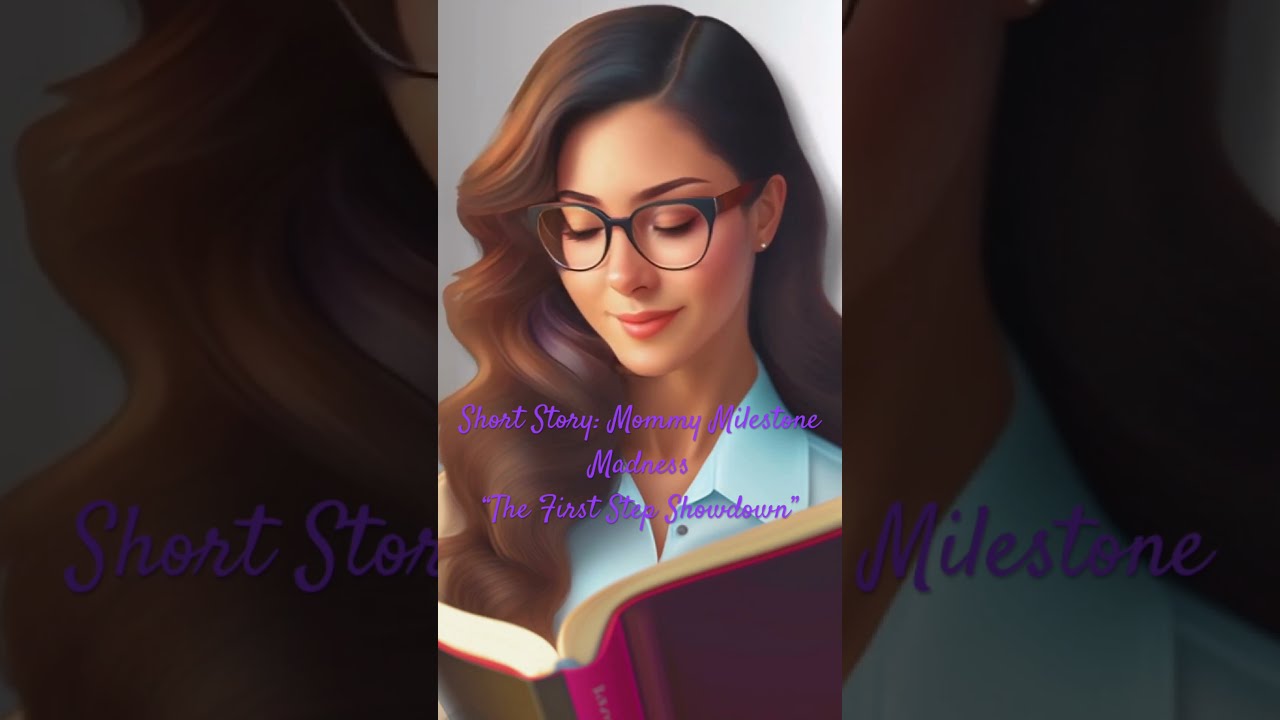This image is a wide rectangular digital artwork composed of three panels. The central panel portrays a woman reading a red hardcover book, labeled in purple font, "Short Story, Mommy Milestone Madness, The First Step Showdown." The woman is depicted from the torso up, wearing a slightly unbuttoned blue collared shirt. She has very long, wavy brown hair with lighter highlights cascading over her shoulders, light brown skin, dark brown eyebrows, and red lipstick on her closed smiling lips. She wears glasses and gazes down at the book. The left and right panels are close-up, darker-shaded images of the left and right sides of the central image, respectively, emphasizing the intricate details of her hair, glasses, and overall presence. The entire piece blends the elements of digital art and watercolor painting, creating a visually captivating scene of tranquil reading.